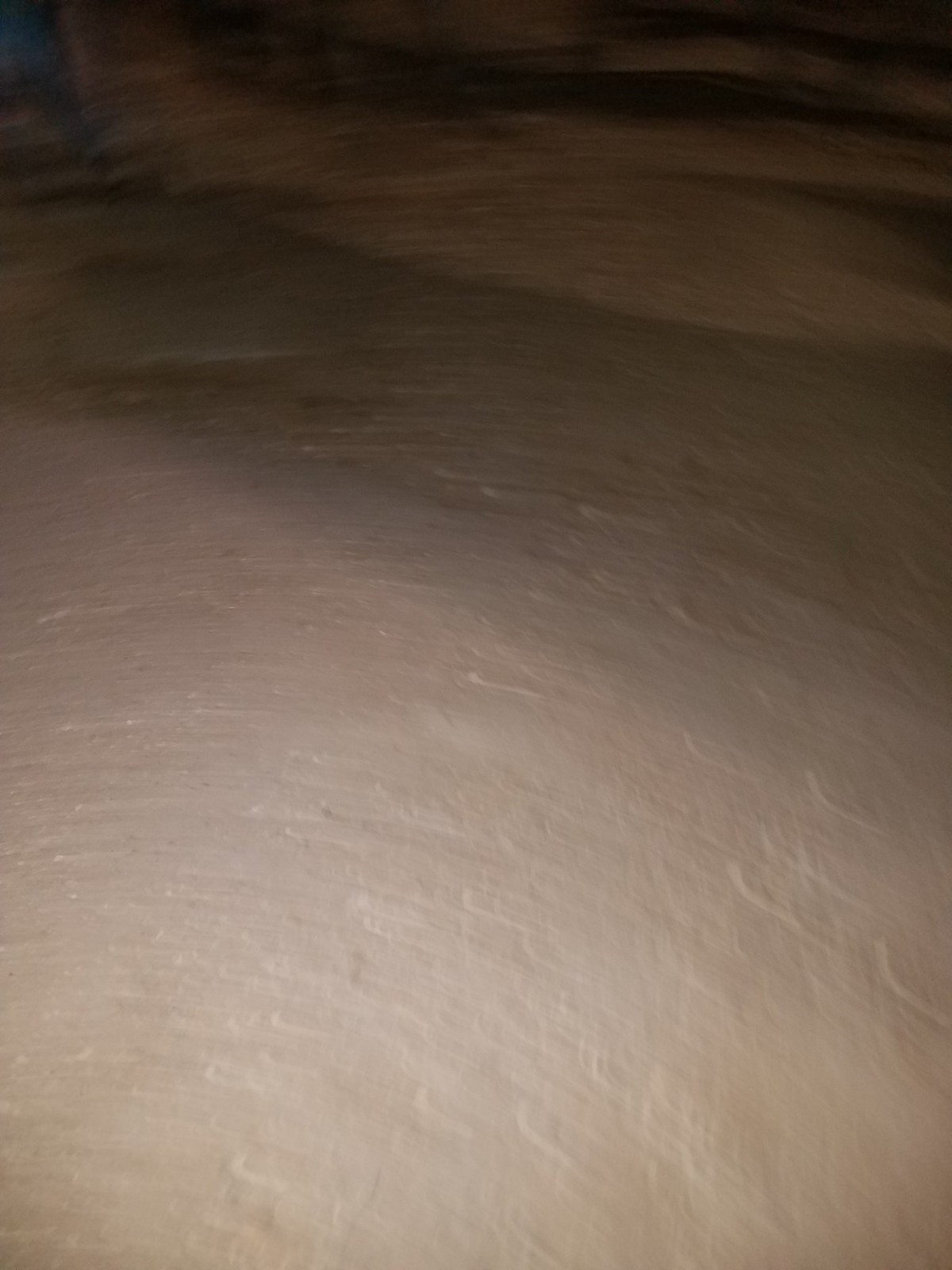In this enigmatic image, the viewer is presented with a scene that is challenging to decode. A snowy landscape seems to be the most plausible interpretation, marked by the presence of indistinct footprints trailing through the snow. The surface, ostensibly white, exhibits subtle tinges of brown or gray, likely the result of lighting effects. The backdrop features a dark horizon, suggesting it is nighttime, with the brighter foreground contrasting against the dim background. Alternatively, it's conceivable that the scene depicts a white brick stone wall, although the lack of distinct contextual clues makes this interpretation less certain. The image’s ambiguity is heightened by the play of shadows and light, creating an atmosphere of mystery and intrigue.